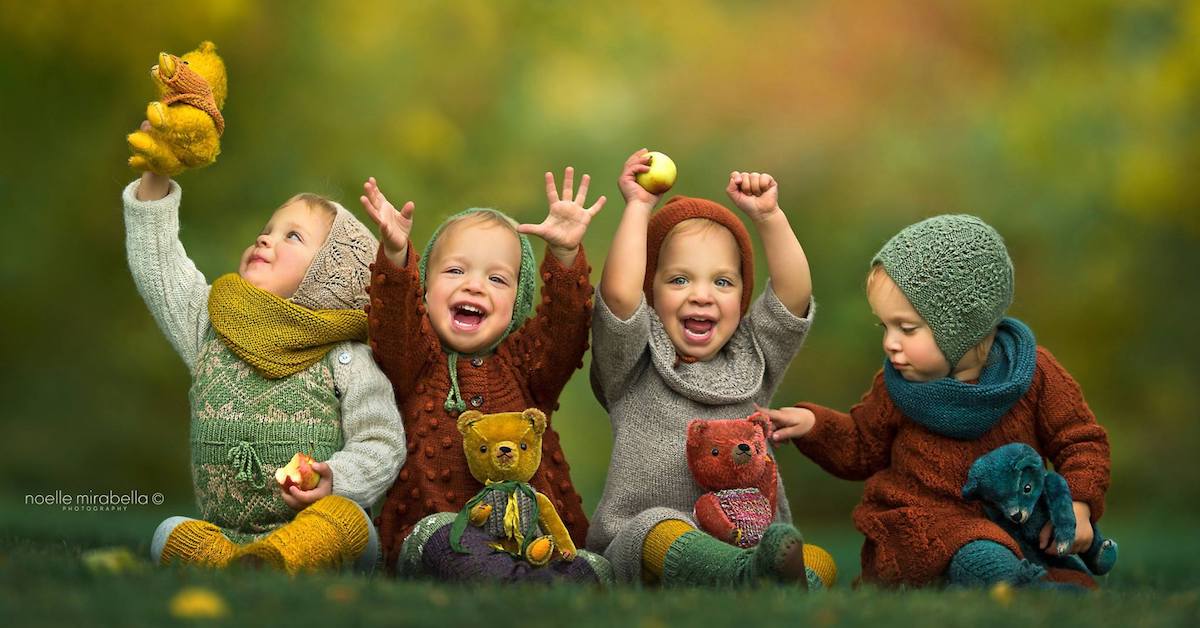In this high-resolution photograph, captured by Noella Mirabella Photography, we see four children sitting on a grassy area, all enjoying themselves and interacting with teddy bears. The children are arranged in a row, each dressed in winter clothing that includes sweaters, scarves, and head coverings. On the left, a child in a green and light blue jersey is holding a yellow teddy bear up in the air while looking at it, with a half-eaten apple in his other hand. Next to him, a child in a brown sweater is joyfully smiling with his hands raised, holding a yellow teddy bear in his lap. To the right, another child in a grey sweater, also smiling broadly with hands up, has a brown teddy bear in his lap and an apple in one hand. On the far right, a child in a brown sweater and blue scarf holds a blue teddy bear and is touching the brown teddy bear in the lap of the previous child. The green grass on which they sit contrasts with the blurred background that features green, yellow, and red hues. Overall, the image captures a moment of happiness and play, with a strong emphasis on the teddy bears each child is holding.